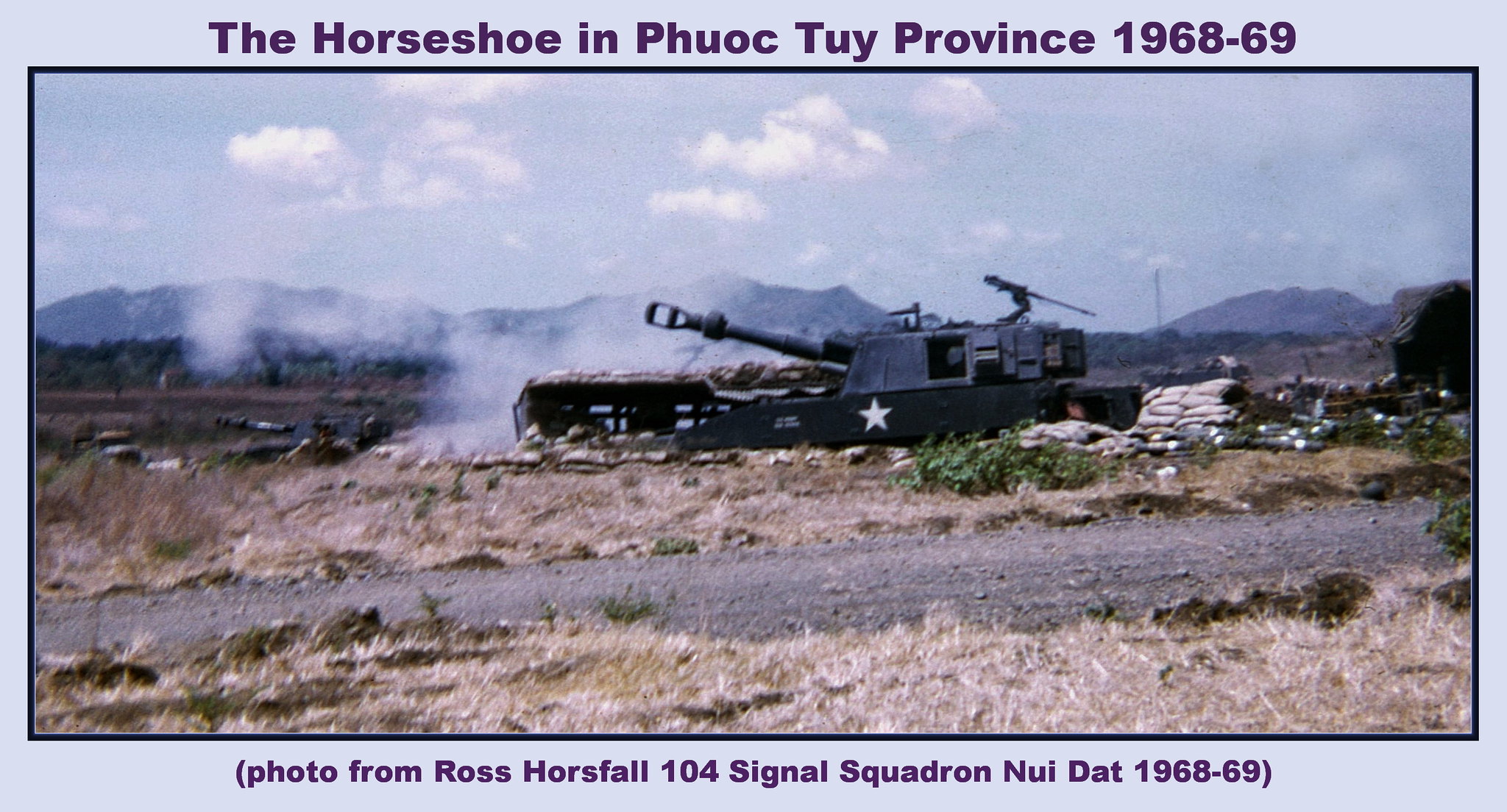This photograph, tinted with a lavender hue, captures a scene from the Vietnam War, specifically titled "The Horseshoe in Phuoc Tuy Province, 1968-69." At the forefront, a black tank adorned with a prominent white star stands in the middle of a dry, sparsely grassed countryside. Billowing smoke emanates around the tank, indicating recent movement or action. In the foreground, a dirt road winds across the scene, while green shrubs and sandbags are visible beside the tank. The sky above is clear and blue, with distant mountains stretching across the background. The bottom of the image bears a caption in parentheses, "Photo from Ross Horsefall, 104 Signal Squadron, Nui Dat, 1968-69," adding historical context to this vivid snapshot.